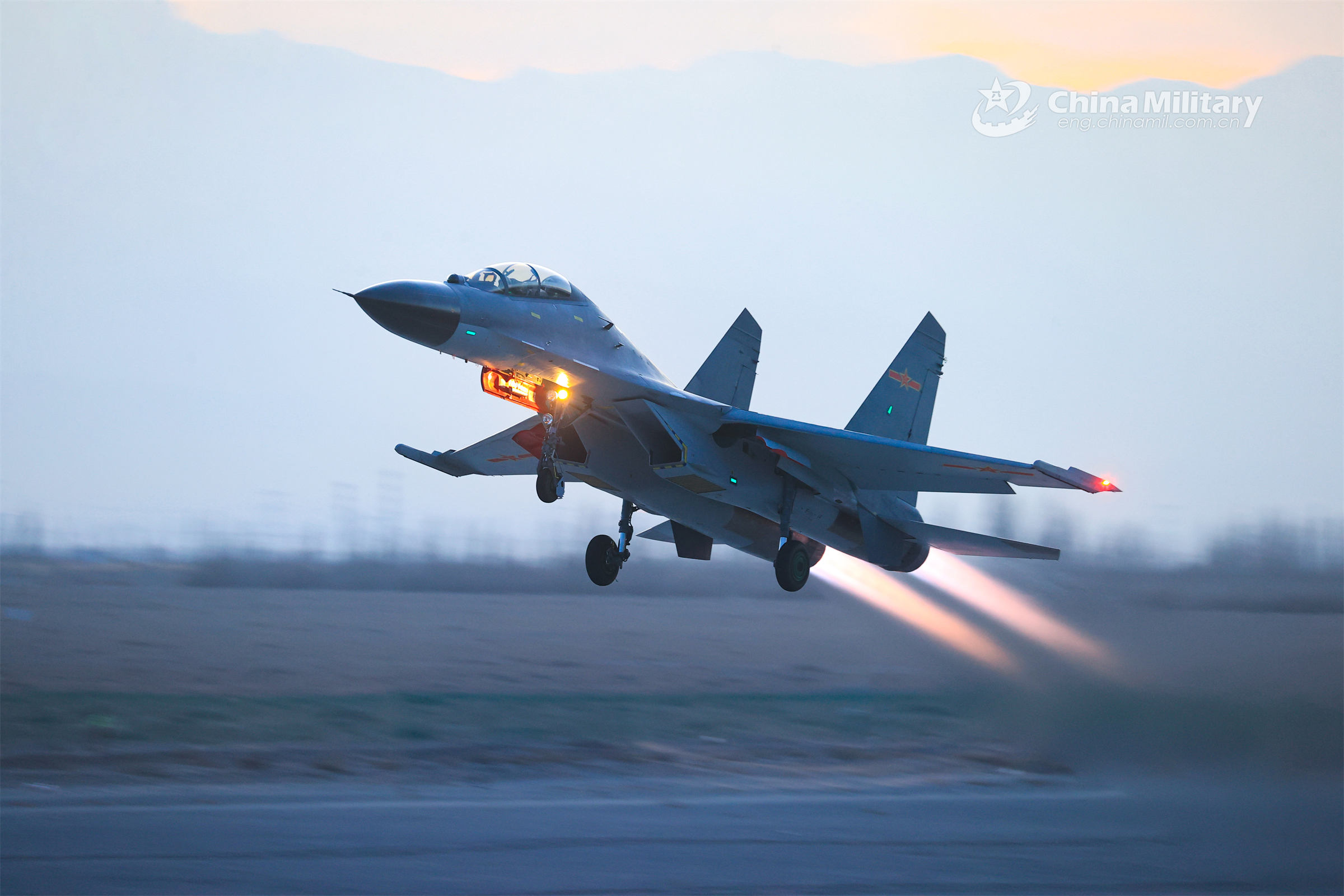The image depicts a small, white or cream-colored Chinese military fighter jet taking off from a barren runway in an open, dirt field. "China Military" along with a star and swirling symbols is prominently displayed in the top right corner of the picture. The jet, which is built for one or two occupants, emits a trail of fire from its rear as it rapidly ascends. It has distinctive features such as a bright yellow-blonde light on its underside, three wheels that appear to be retracting, and a total of six wings—two main wings and two smaller sets at the rear. The scene is set against a cloudy, gray sky, suggesting early morning or late evening conditions.